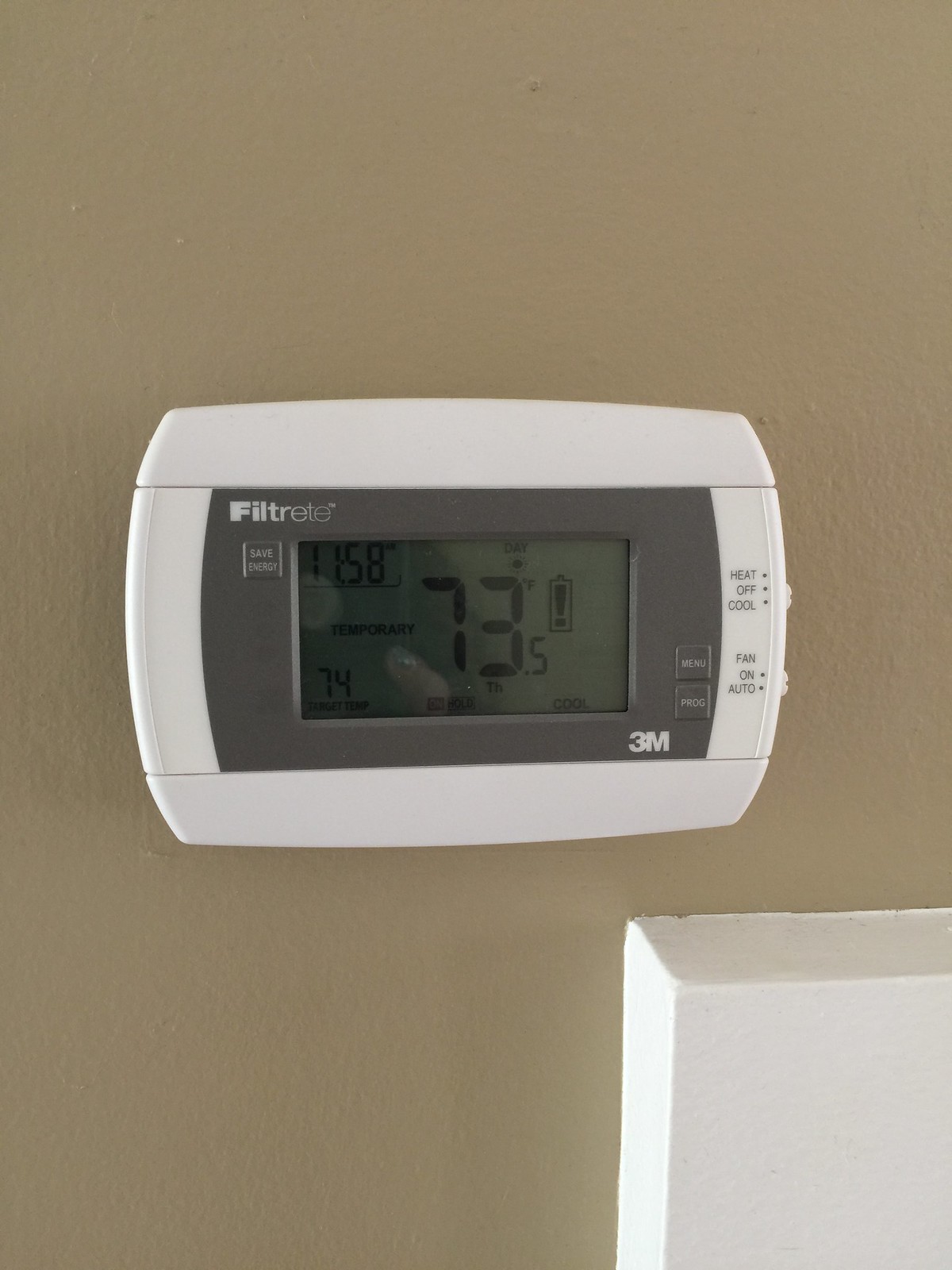The photograph displays a thermostat affixed to a slightly textured, tannish light brown wall. In the bottom right corner of the image, a white object with a corner protruding from the wall is visible, though its exact purpose remains unclear. 

The thermostat itself has a predominantly rectangular shape with curved edges and features white sides. Embedded within this white casing is a grey rectangular display area. At the top left of this grey section, "Filtrete" is prominently displayed, followed by a "Save Energy" button directly below it. On the right side of the grey area, two additional buttons are labeled "Menu" and "Prog." Further down, the brand name "3M" is printed in white.

To the right of the many buttons and indicators in the grey section, the white casing features labels for "Heat Off Cool" and "Fan On Auto" along with corresponding small switches for these settings. 

The digital readout on the thermostat displays a current temperature of 73.5 degrees Fahrenheit. A digital thermometer icon with an exclamation mark is present, indicating a possible issue or alert. The display also shows that it is currently "Day." At the bottom of the display, "Target Temps" is noted, with a target temperature set at 74 degrees. The thermostat is in "On" or "Hold" status, with an indicator showing that it is Thursday. The system is set to "Cool" mode. In the upper left corner of the display, the current time is shown as 11:58 AM.